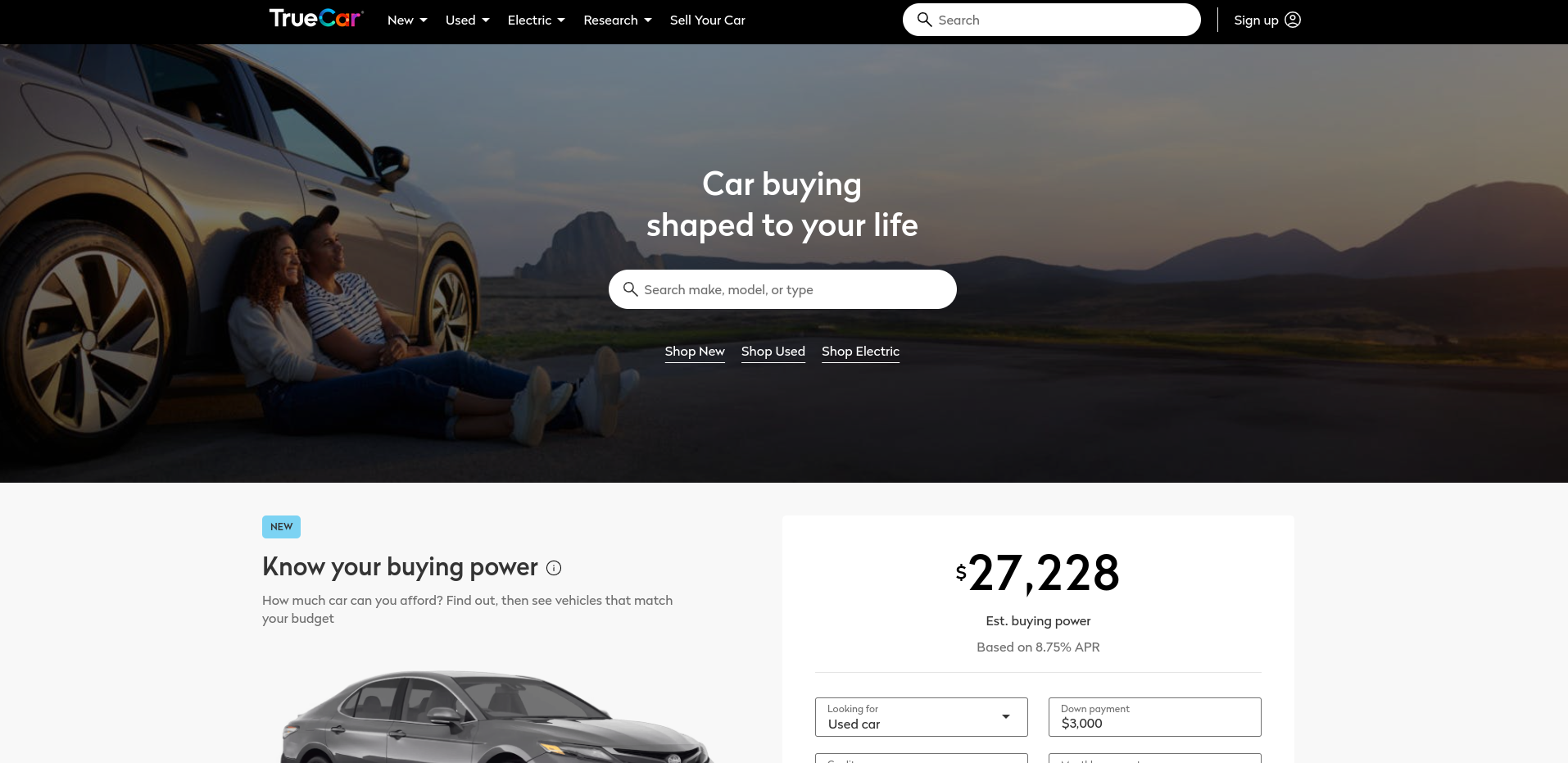This is a screenshot from the TrueCar website, a platform for buying and selling cars. The top of the screenshot features a black strip containing the TrueCar logo, positioned about one-fifth of the way from the left. The word "True" is displayed in white text, while "Car" is in multicolored letters, with "C" in green, "A" in red, and "R" in orange. 

To the right of the logo, there are five tabs: "New," "Used," "Electric," "Research," and "Sell Your Car." Also situated along this black strip is a white search bar with a magnifying glass icon on its left side and the prompt "Search." On the far right of the search bar is a "Sign Up" button.

Beneath this top strip is a large banner photograph depicting a young man and a young woman sitting on the ground, leaning against the side of a shiny car. They are on a road that winds towards a distant mountain range. The accompanying text on the banner reads, "Car buying shaped to your life."